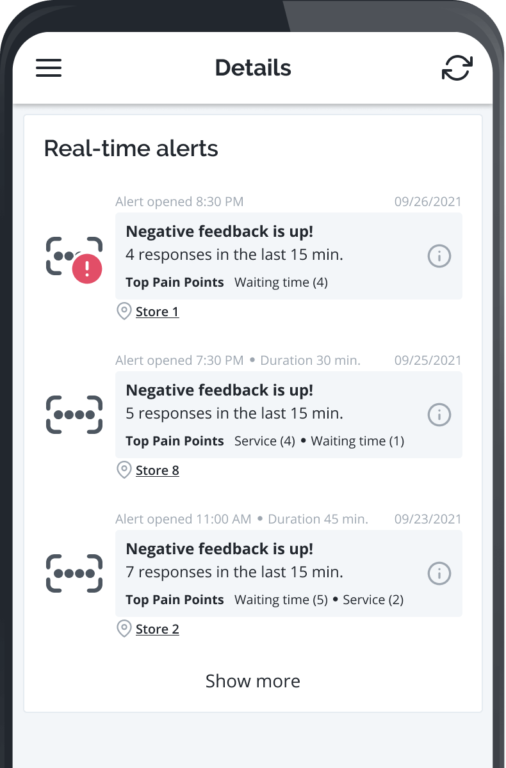This image showcases a mobile device with a black frame. The display screen features a white background. In the upper left corner, there is a list button, while the upper right corner houses a refresh symbol. Centrally located on the screen, the word "Details" is prominently displayed in black letters.

Below the title, the content is organized into detailed notifications starting on the left side:
1. The first alert reads: "Real-time alerts".
   - "Alert open: 8:30 p.m. on the 26th of September 2021".
   - It indicates a trend: "Negative feedback is up by 4 responses in the last 15 minutes".
   - Top pain points specified are: "Waiting time for Store One".

2. The subsequent notification reveals:
   - "Negative feedback is up by 5 responses in the last 15 minutes".
   - Highlighted issues include: "Service for Waiting Time at Store Eight".

3. The last segment reports:
   - "Negative feedback is up by 7 responses in the last 15 minutes".
   - Crucial concerns are: "Waiting Time for Store Five and Service at Store Two".

At the bottom of the screen, there is a clickable button labeled "Show More".